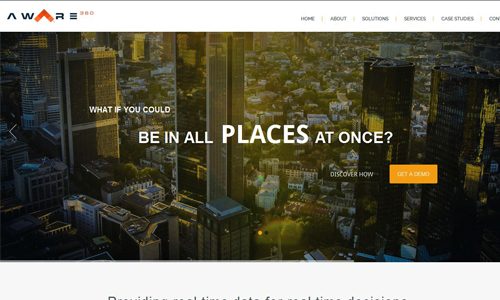A screenshot of a web page is displayed, showcasing a website named "AWARE." The word "AWARE" is styled with a red, upside-down V representing the letter "A," followed by "W-A-R-E" in standard text. 

At the top of the page, there's a navigation bar with drop-down menus labeled "HOME," "ABOUT," "SOLUTIONS," "SERVICES," and "CARE STUDIES," though the last menu item is partially cut off. 

Central to the screen is a captivating image of a sprawling urban landscape, featuring towering, shiny skyscrapers juxtaposed with lower buildings and houses. Overlaying this image, a white text header reads, "WHAT IF YOU COULD," followed by the prominent, larger-font message, "BE IN ALL PLACES AT ONCE?" The word "PLACES" stands out in all capital letters and is the largest word visible on the screen.

Below this bold statement, small white text invites users to "DISCOVER HOW." Beneath this text is an orange button with white lettering that reads "GET A DEMO," offering an interactive element for website visitors.